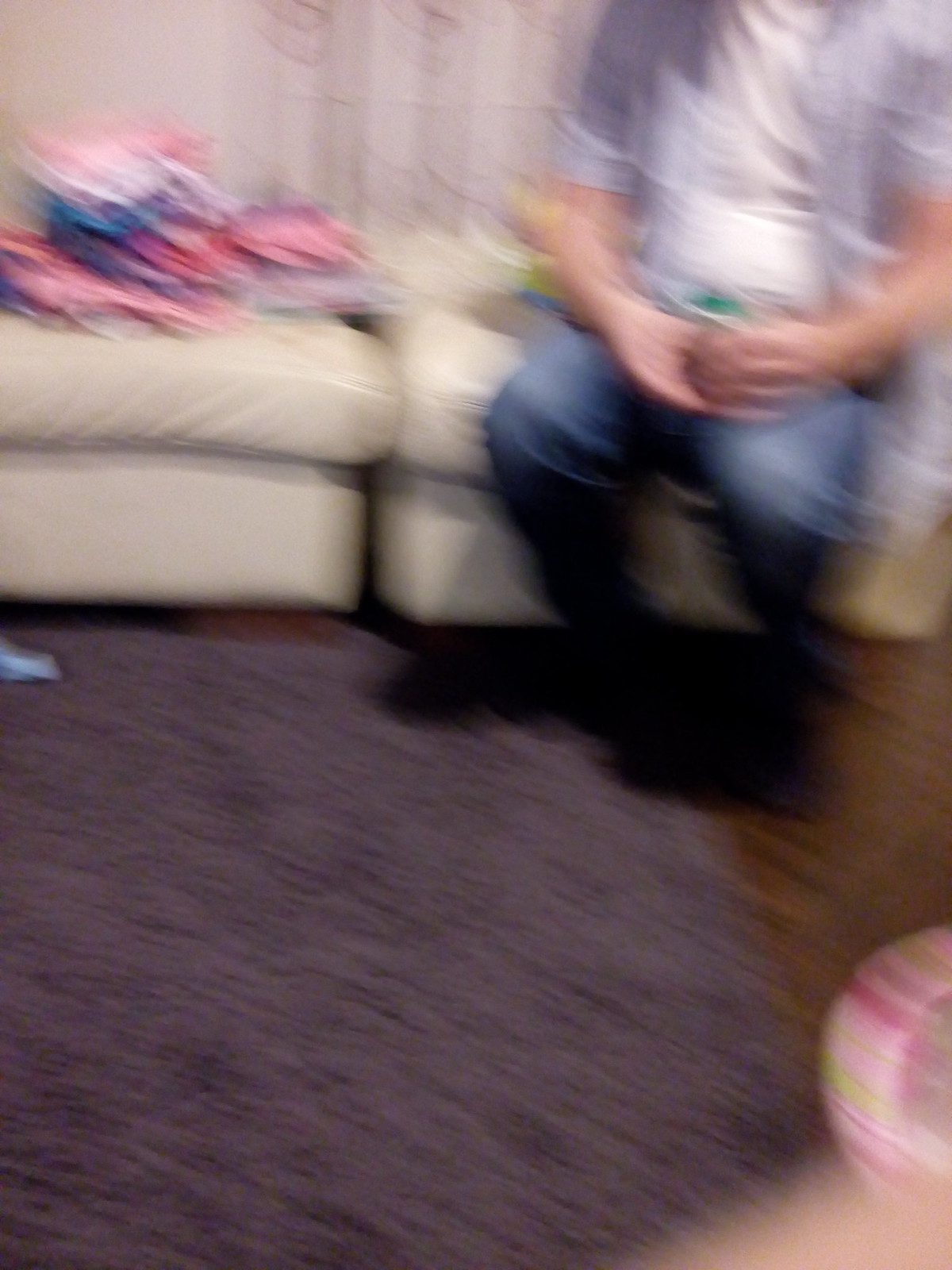This photograph captures a blurred interior scene, likely due to the camera moving during the shot. The focal point is a cozy white sofa laden with numerous white cushions. On the leftmost cushion, several small pink objects are scattered. On the right side of the sofa, a person is seated; they are dressed in a white shirt and blue jeans, with their bare arms visible. At their feet, there's an indistinct black blur that could be another smaller rug. In front of the sofa lies a grey rug with a small blue item placed on it. The room features a patch of brown to the right, possibly indicating wood flooring. In the foreground, the bottom right corner of the image reveals a pink object with stripes, the nature of which is unclear due to the overall blur.